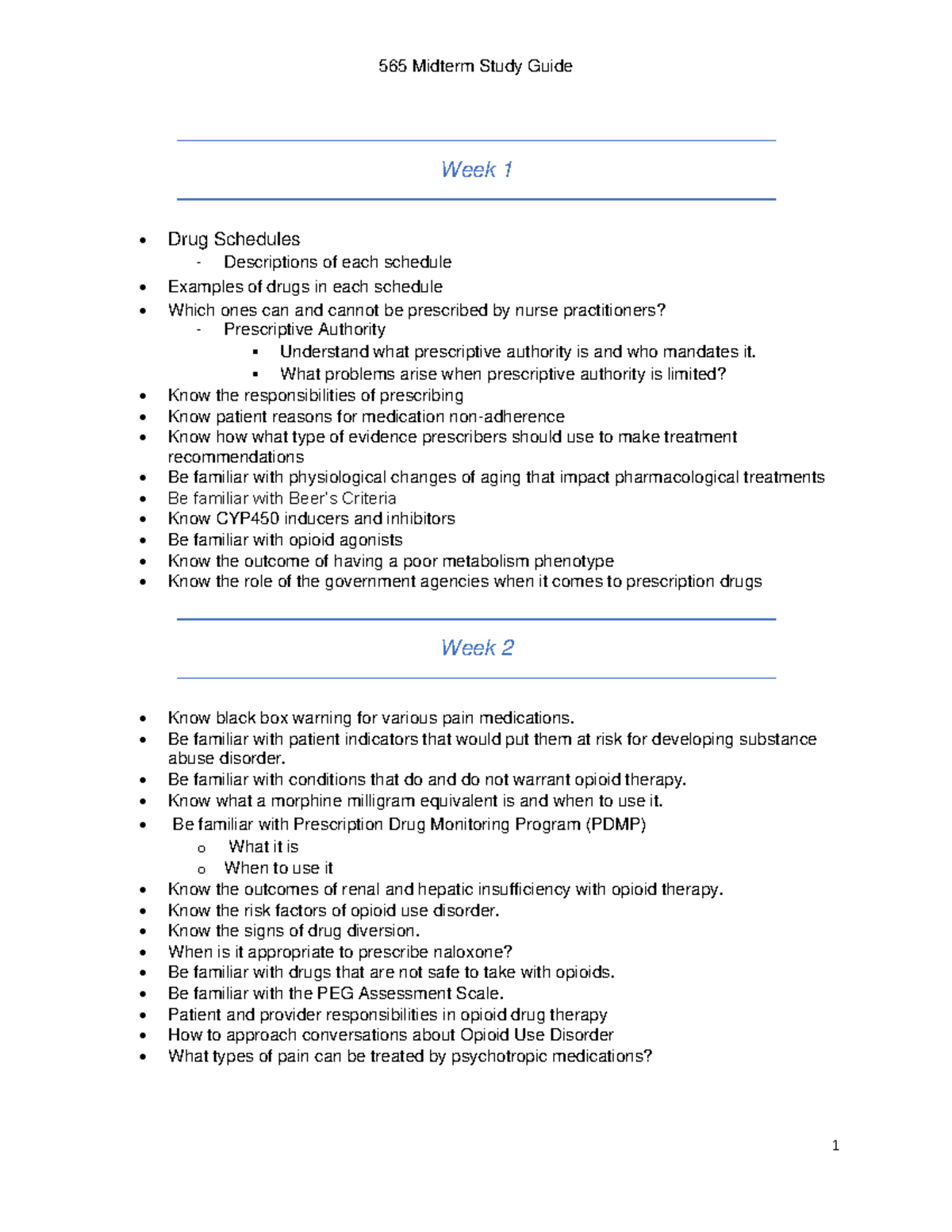The image depicts a detailed breakdown of an "MS5 Midterm Study Guide." At the top, the title is prominently displayed with the text "MS5 Midterm Study Guide" followed by a thin blue horizontal line. Below this header, the guide is divided by weeks.

For "Week One," centered blue text marks the section, underscored by another thin blue horizontal line. This section features a list of 15 bullet points detailing key topics such as drug schedules and examples of drugs corresponding to each schedule.

Following the week one content, another thin blue horizontal line separates the sections. The "Week Two" section begins with its title centered in blue text, also underlined by a thin blue line. This section contains 14 bullet points, each detailing essential information, primarily in black text. Examples of the content include notes stating "No black box warning for various pain medications," advisories to "Be familiar with patients and the factors that put them at risk for developing a substance abuse disorder," guidelines on "Conditions that do or do not warrant opioid therapy," and explanations about "Morphine milligram equivalents and when to use them."

Overall, the study guide is organized and structured to provide a comprehensive overview of critical topics for the MS5 midterm, presented in a clear and detailed manner.